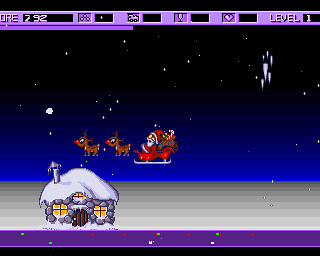A nostalgic screenshot of a retro-style video game, likely designed for PC, set against a black backdrop that emulates a night sky illuminated by a subtle blue light on the horizon. The stars are depicted as tiny dots scattered across the sky. Dominating the scene, Santa Claus rides in a sleigh, holding a brown backpack and a candy cane, pulled by two reindeer, each featuring a distinctive red nose. Below, a quaint stone cottage covered in snow serves as the focal point of the terrestrial setting. The cozy house, detailed with three windows and a wooden door, features a small chimney protruding from the roof. The snowfall, represented by small white dots, gently descends, blanketing the ground in a layer of snow, adding to the wintry atmosphere of the image.